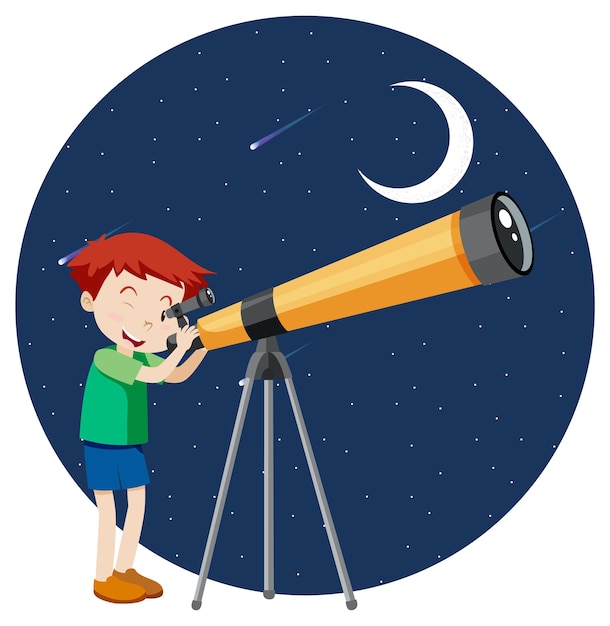This detailed digital drawing features a cartoon-like image of a joyful boy with fair skin and red hair, standing within a stylized circular border representing the night sky. The circle, which forms the backdrop, is filled with blue hues, white stars, and a crescent moon facing left. Additionally, three shooting stars (or comets) add dynamic elements to the celestial scene. The boy stands on the left, dressed in a green shirt, blue shorts, and brown shoes, and is looking through a yellow and black telescope mounted on a gray tripod. His red eyebrows and expressive face, with one eye closed and the other gazing through the telescope, convey his fascination with stargazing. This charming artwork captures the wonder and excitement associated with astronomy.